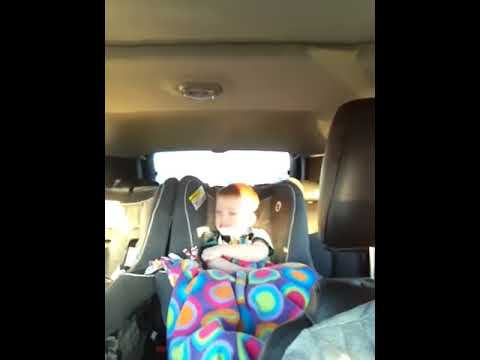The photograph, framed with vertical black borders making it taller than wide, captures an interior view of a car during the daytime. The perspective is from the front seat, looking back. Central in the image is a young Caucasian boy, around 8 months old, seated in a gray car seat. The baby, with short reddish hair, is looking toward the camera but has his face turned slightly to the left, seemingly reacting to sunlight coming from the right side. The child is wrapped in a multi-colored blanket adorned with blue, orange, pink, yellow, green, white, and purple blobs. Above the child, the car's beige or off-white ceiling is visible, and below, there's some detail of a headrest and the shoulder of an individual in the front seat, wearing a light blue top. Light filters through the rear window, contributing to the soft illumination of the scene. A marker or label is affixed to the child's seat, though it is too distant to read.